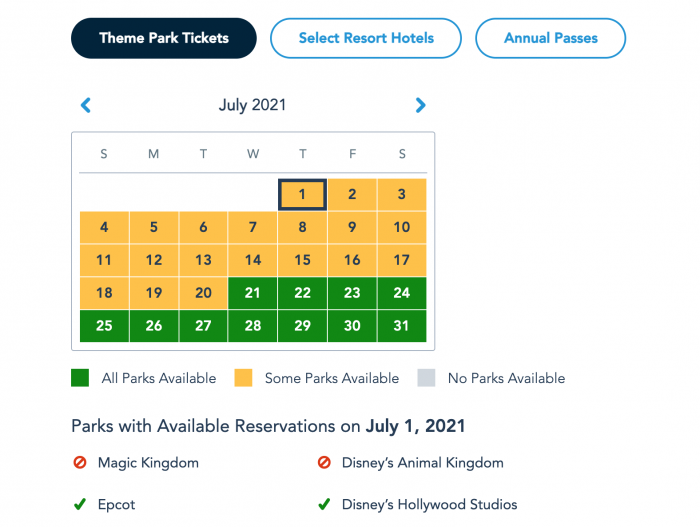**Detailed Descriptive Caption:**

The image appears to be a screenshot from the Disney website with a white background. In the top left corner, there's a dark blue oval button with white text that reads "Theme Park Tickets." To the right of this button, there is a white oval button outlined in blue containing blue text that says "Select Resort Hotels," followed by another similar button with blue text that reads "Annual Passes."

Beneath the "Theme Park Tickets" button, there is black text displaying "July 2021," flanked by blue arrows pointing left and right. Below this, a calendar for July is shown. The days of the week are listed in light green text across the top, starting from "S" for Sunday on the far left, followed by "M, T, W, T, F," and ending with "S" for Saturday on the far right. 

The dates begin on the row under the "T" for Thursday and "F" for Friday, starting with the 1st in a yellow box. All dates from the 1st to the 20th are in yellow boxes. The 20th is a Tuesday, and the next day, the 21st, is marked with a green box indicating Wednesday. The dates continue in yellow boxes until the month ends on the 31st, a Saturday, at the bottom right of the calendar.

Under the calendar, there are three colored boxes. The first box on the left is green with light gray text that says "All Parks Available." The middle box is yellow with light gray text that reads "Some Parks Available." The box on the right is light gray with text that says "No Parks Available."

Beneath these colored boxes is black text stating "Parks with Available Reservations on July 1, 2021." Listed below this title, arranged in two columns, are the names of the parks. On the left column, it lists "Magic Kingdom" and below that, "Epcot." In the right column, next to "Magic Kingdom," it lists "Disney's Animal Kingdom," with "Disney's Hollywood Studios" listed underneath.